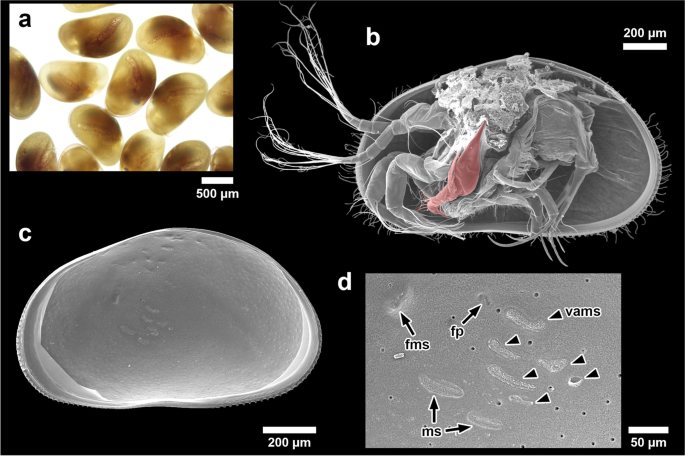The image comprises four detailed panels labeled A, B, C, and D, all set against a black background. Panel A features what appear to be yellow, slightly translucent, bean-shaped structures, resembling cells or possibly egg sacs. In panel B, a close-up, possibly microscopic, view of one of these structures reveals the presence of something inside that resembles an insect or bug, potentially a flea, with legs visible. The scale indicator in the upper right suggests a measurement, likely in nanometers. Panel C presents the bean-shaped structure again, but this time without the internal details, giving a solid appearance. Finally, panel D showcases the structure within a microscopic view, annotated with various abbreviations such as FMS, FPMS, and VAMS, indicating different labeled points of interest. The overall color palette is predominantly grey with accents of pink and yellow, suggesting a scientific investigation, possibly into a biological system infected with a virus or bacteria.